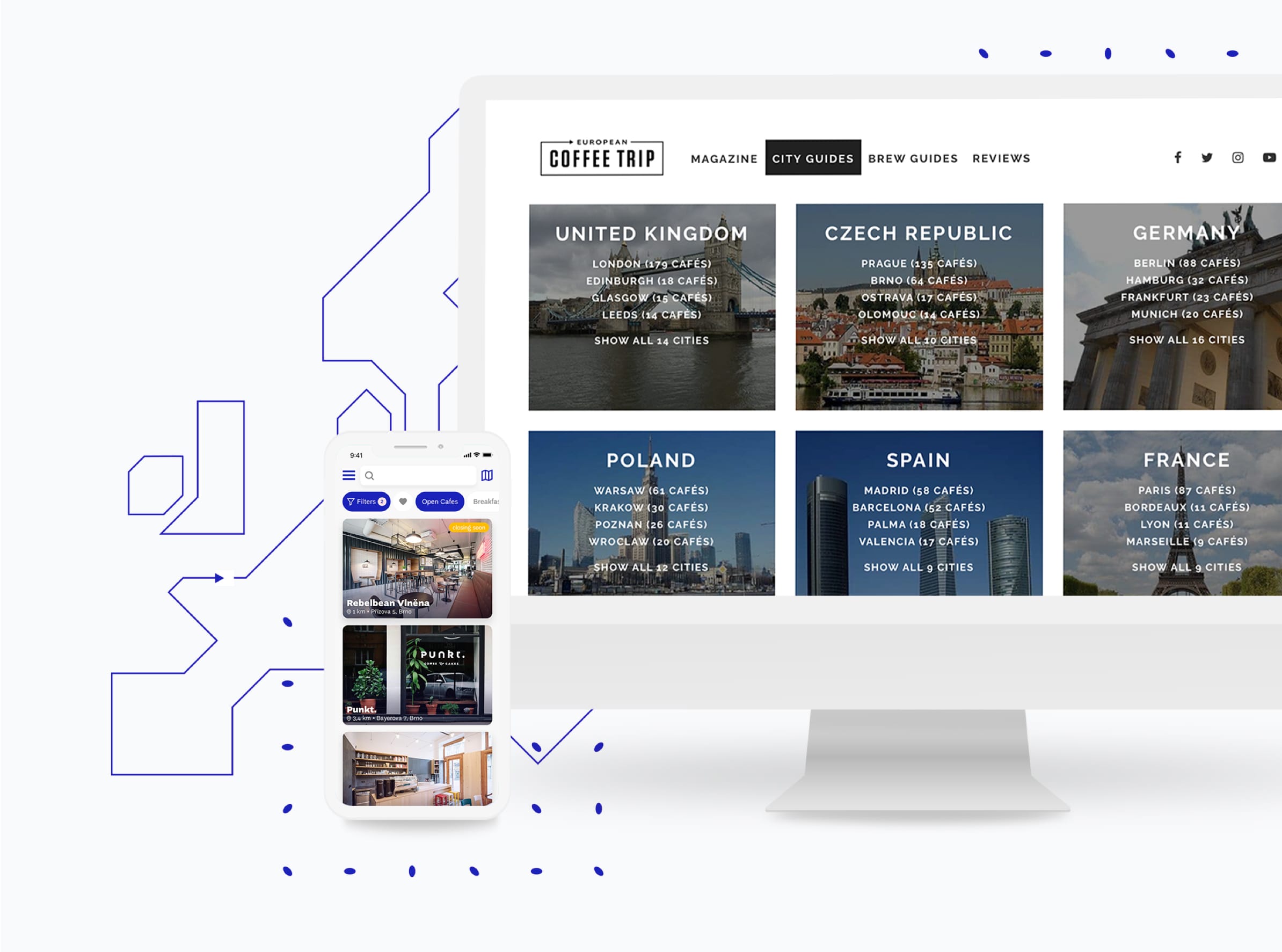This image showcases a clean, modern website with its interface displayed side-by-side on both a computer monitor and a mobile phone. Both devices are encased in sleek, white borders, contributing to the overall minimalist aesthetic. The left side of the image features a whimsical purple design composed of various geometric shapes and small dots, adding a playful touch.

The website highlighted is dedicated to European coffee trips, offering comprehensive guides and reviews for coffee enthusiasts. It includes sections for city guides, brew guides, and user reviews. The site provides options to explore the coffee culture in several European countries, including the United Kingdom, the Czech Republic, Germany, Poland, Spain, and France. Each country is presented in its own neatly organized box, adorned with stunning background images depicting relevant scenic locales.

A key feature displayed on the mobile phone is a list of open cafes, showcasing different establishments available for visit. Noteworthy mentions include "Rebel Bean Veneer," which appears to be a charming eatery, and "Punk C," highlighted for its inviting windows and lush greenery. Another spot is depicted with a view of a cozy interior, featuring a countertop, chairs, and shelves, indicating a welcoming place to enjoy coffee.

The website's design maintains a crisp, white background, enhancing readability and navigation. Social media icons for Facebook, Twitter, and Instagram are conveniently located on the right side of the computer monitor, inviting users to explore more and stay connected. Overall, it's a fascinating and user-friendly guide for anyone planning a coffee adventure across Europe.